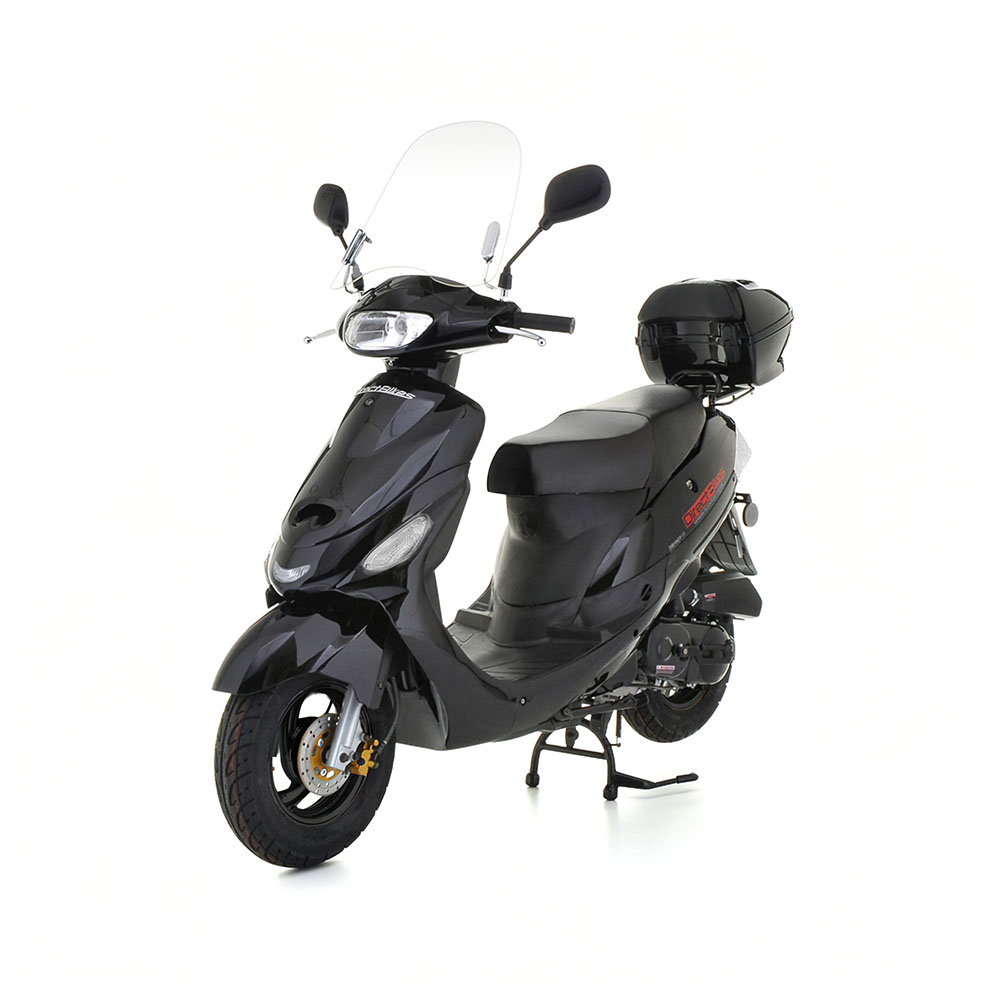In this image, set against a completely white background, there is a black electric scooter, resembling a moped. The scooter, positioned so that the front wheel is pointed towards about 7 o'clock, features a sleek, matte black body that is shorter and thinner compared to a traditional motorcycle. Both the front and back wheels are a darker shade of black, complementing the black frame and body. The scooter stands upright on its rubbery kickstand located underneath.

On the rear right side, just behind the seat, a red-colored brand name "Direct Bikes" is visible, although partially hidden due to the angle of the shot. The seat itself appears smooth and leathery. Attached to the back is a small black luggage container, often used for storing items like a helmet.

The front of the scooter sports a small windshield and a set of four headlights—one on the handlebars and three positioned just above the front wheel. Black rearview mirrors flank either side of the steering column, which includes the throttle, brake levers, and controls. Silver brakes add a slight contrast to the otherwise entirely black color scheme.